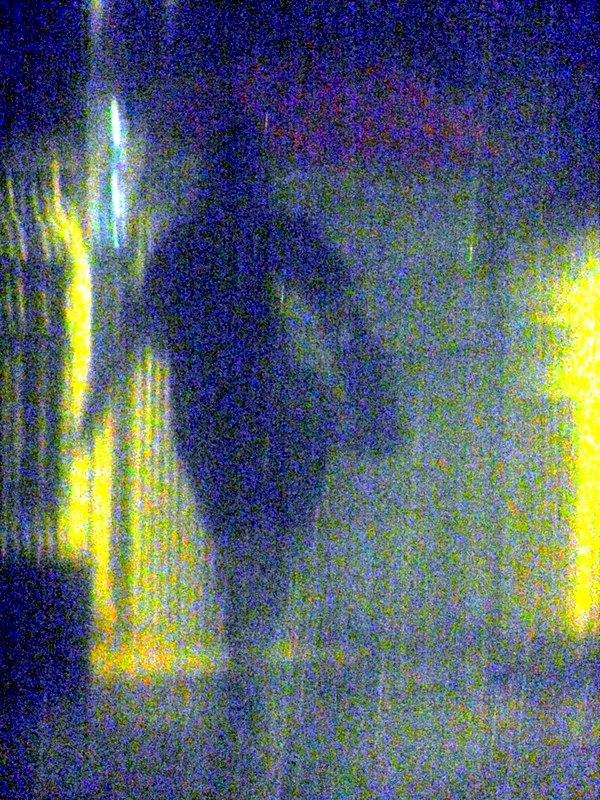In this pixelated and abstract photograph, the central focus is a silhouette of a person, set against a predominantly dark background. The majority of the image is enveloped in deep black, creating a stark contrast that emphasizes the silhouetted figure. Along the right edge, a striking band of yellow and white adds a vibrant touch, which gradually transitions into a mesmerizing bluish-purple-green pattern. This colorful gradient snakes through the darkness and re-emerges as another band of yellow and white on the other side of the silhouette. To the left, a series of squiggly lines add a detailed, almost whimsical element, further enhancing the mysterious and artistic nature of the photograph.